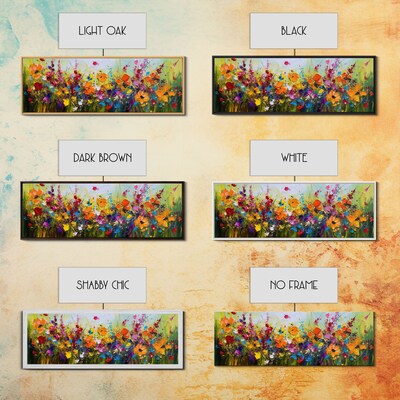The image, a detailed illustration, showcases a vibrant floral artwork surrounded by various types of frames to demonstrate framing options. Set against a blended backdrop of brown, cream, orange, and a hint of blue in the upper left, the square image features six examples arranged in two columns. Each floral pattern, blooming in a spectrum of rainbow colors, is framed distinctly to highlight different styles: the first column from bottom to top displays options without a frame, with a white frame, and with a black frame; the second column shows the same floral image framed in shabby chic (white with a black overlay), dark brown, and light oak. Above each framed picture, a corresponding rectangular box labels the frame color, helping viewers visualize the contrast and effect each frame style provides. This visually rich setup elucidates how different frames can enhance or alter the perception of the artwork.